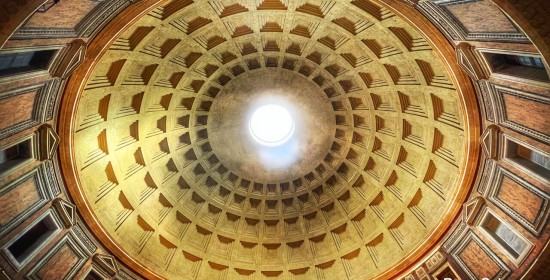This photograph captures the interior dome of a building, possibly a luxurious hotel, government building, or even the Pantheon in Rome. Taken from ground level, it showcases a stunning circular ceiling adorned with intricate designs. The dome's lower half features an array of rectangular windows, with those on the left appearing darker than those on the right. Above each window, small triangles accentuate the symmetrical pattern. 

The primary colors in the dome's design are yellow and brown, with the hues intensifying as they ascend towards the center. This creates a gradient effect that culminates in a copper-colored circle. At the very heart of this circle is a smaller aperture, which allows natural sunlight to stream into the room below, creating a mesmerizing focal point reminiscent of an eye looking down. The overall design is not only strikingly beautiful but also conveys a sense of depth and three-dimensionality, enhanced by the interplay of light and shadow.